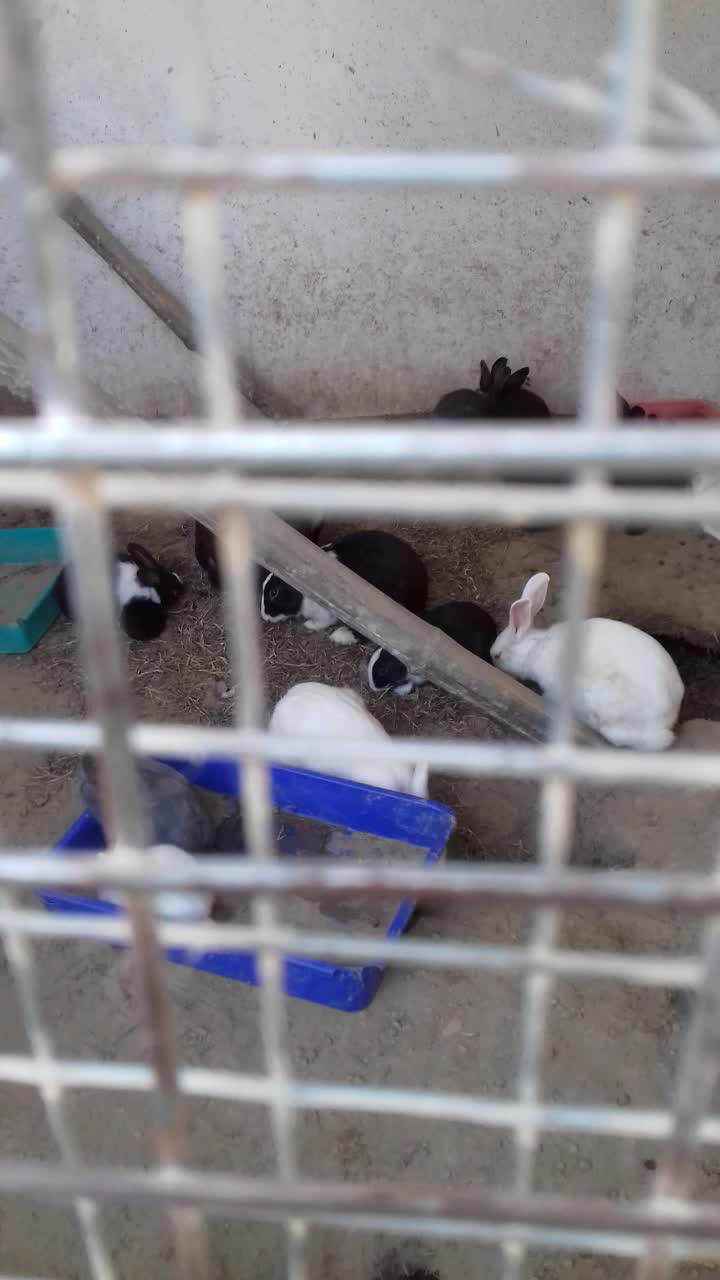In this outdoor photograph, captured through the blurry metal grid of a cage, the scene focuses on a group of adult rabbits within a penned area. The cage's square metal bars frame the image, partially obscuring the foreground. Inside the enclosure, the rabbits rest, sleep, or nibble on something on the dirt floor scattered with rocks and hay. The central focus reveals eight to nine rabbits of various colors: primarily black with white splotches, pure white, and solid black. Notably, there is a blue litter box, in which a gray rabbit appears to be sitting, and a light greenish bucket, both likely containing clay. In the background, a grimy concrete wall, once white but now stained, suggests a utilitarian setting. Overall, the composition captures a moment of calm in the rabbits' daily life.